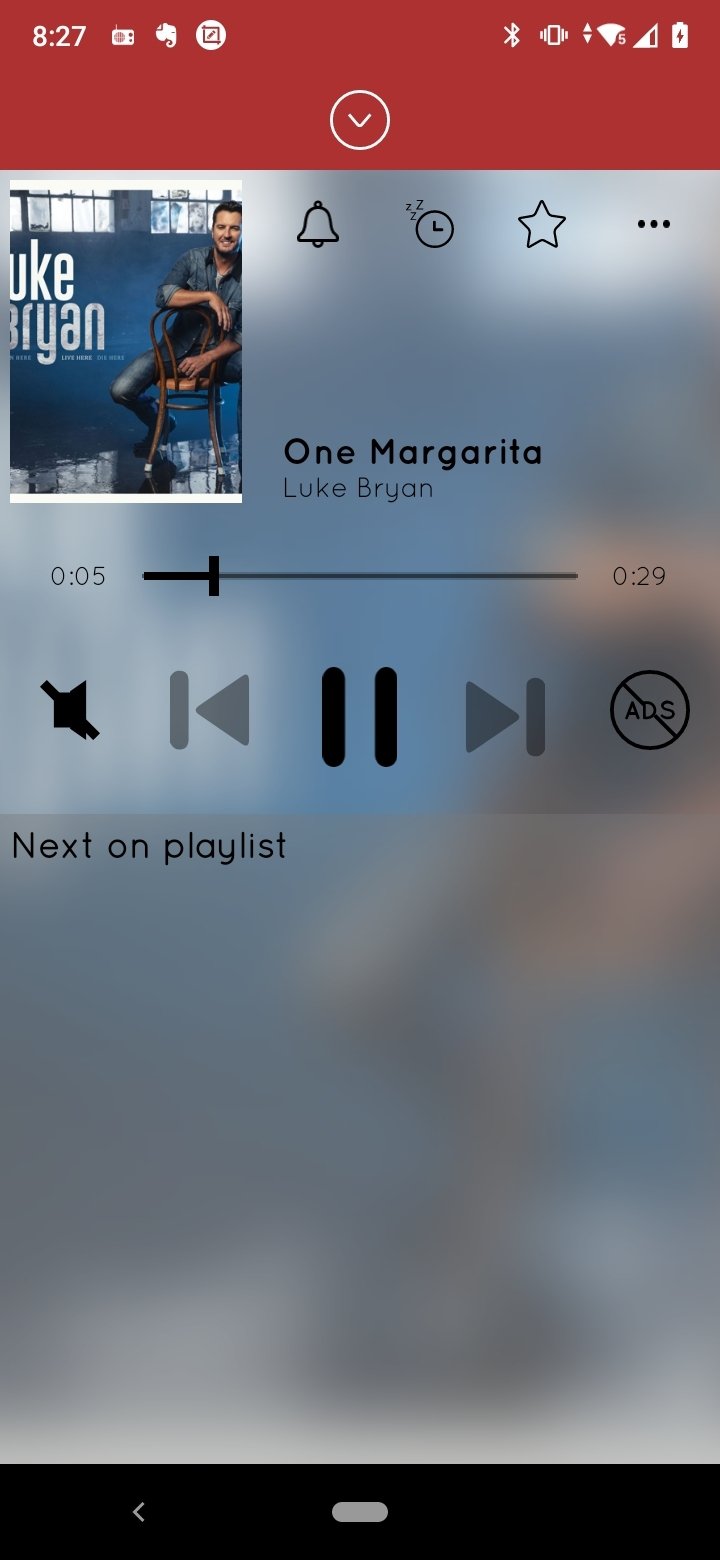The screenshot of the device displays various status indicators and notifications on the screen. In the top-left corner, the time is shown as 8:27 alongside a radio notification icon. The top-right section features multiple icons including Bluetooth, vibration mode, a Wi-Fi signal, a network signal bar, and a battery charging indicator. Just below these icons, there is a drop-down arrow for additional options.

An alarm notification bell icon is visible, next to which there are icons for a set timer, markers, and favorites. The music player interface is prominently displayed, showing that "One Margarita" by Luke Bryan is currently playing, five seconds into a 29-second playlist, although the sound is inactive. The interface includes controls for the previous track, play/pause, and the next track.

At the bottom of the screen, the navigation keys are present, including the back key and the home key, providing easy access to essential functions.